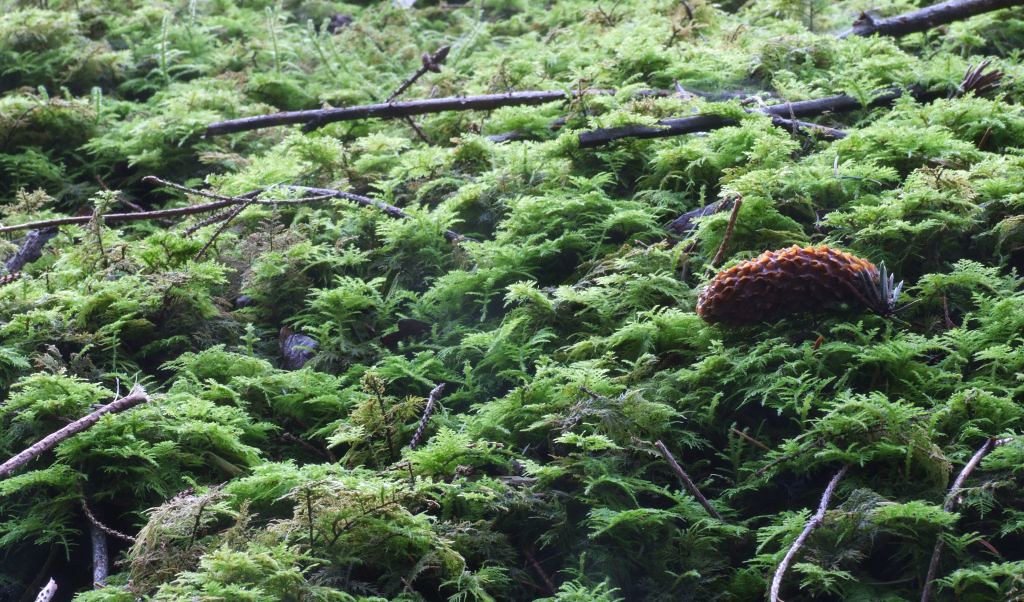This photograph, taken in a lush, outdoor natural setting during the daytime, showcases a vibrant, healthy environment rich with plant life. The scene is predominantly filled with green leaves, indicative of a thriving forest or rainforest canopy. Scattered throughout the dense greenery are several tree branches, some dark brown and others possibly black, lying both vertically and horizontally as if some have fallen. In the right mid-ground of the rectangular, landscape-oriented image, there is a notable orange and brown object—it could be a caterpillar, a pine cone, or some type of seed-bearing structure—sitting atop the foliage, adding a point of interest amid the verdant backdrop. The photograph captures the intricate details and textures of the forest floor, with elements of moss, grass, and potential weeds enhancing the natural, untamed beauty of the scene.